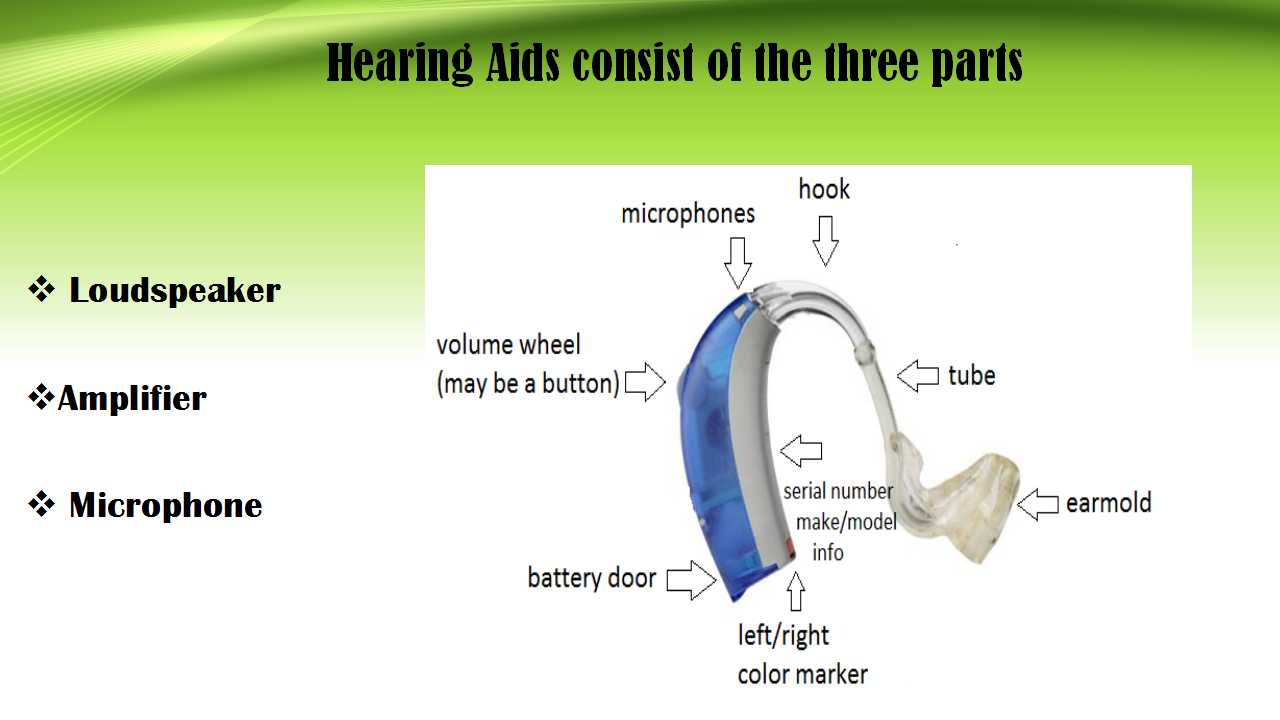This image is a detailed diagram of a hearing aid, presented in a side view and formatted like a PowerPoint slide. The top of the page features a green heading that reads "Hearing Aids Consist of Three Parts," in reference to the loudspeaker, amplifier, and microphone, which are listed in black lettering in columns on the left-hand side. 

At the center of the diagram, inside a white cut-out square area, there is a depiction of a blue and gray hearing aid, with transparent plastic parts, and black labeling with arrows pointing to its various components. The labeled parts include the microphone at the top, a hook adjacent to it, a volume wheel on the curved portion alongside a possible button, and the battery door at the bottom. Other arrows point to the ear mold, tube, and a left to right color marker on the right-hand side. Additionally, the make, model info, and serial number are identified on the hearing aid in the diagram.